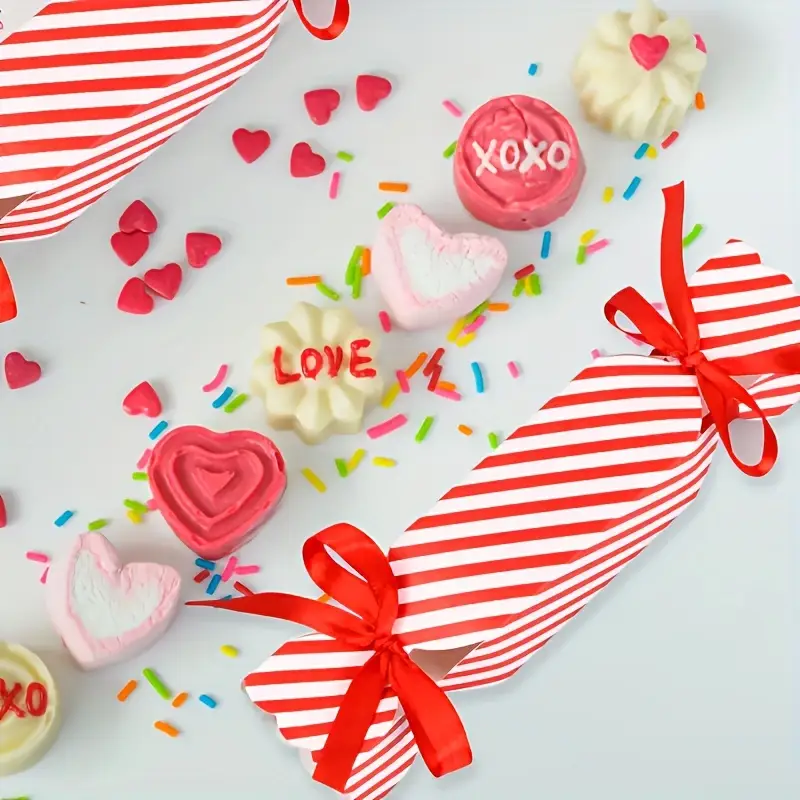The image features a meticulously arranged display, primarily set against a light gray background. Central to the composition are two rectangular packages, adorned with red and white striped wrapping paper, each tied at both ends with red bows. Scattered around the packages are various candies and treats, vividly evoking a Valentine's Day theme. The candies, resembling little marshmallow-like confections and white chocolates, are decorated with pink hearts and an assortment of colorful cake sprinkles in pink, blue, and green. Among the sweets are several heart-shaped and circular treats, some inscribed with endearing messages such as "XOXO" and "LOVE." The overall arrangement suggests a festive, romantic atmosphere, with a focus on love and affection.